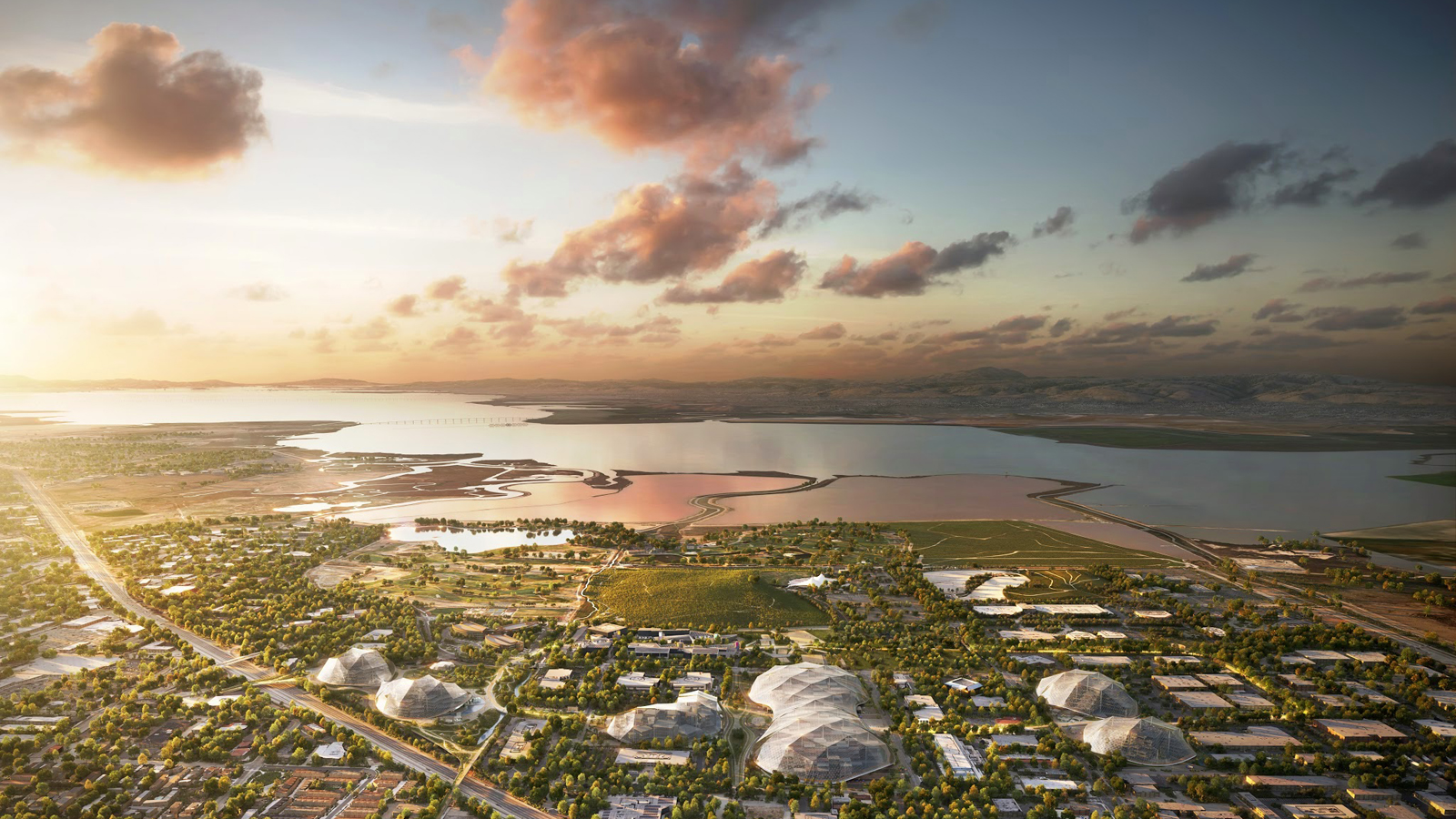This horizontally aligned rectangular aerial photograph captures a serene town scene from a few hundred feet above. The top half of the image showcases a sky transitioning from light to dark with hues of orange, pink, yellow, blue, and white, reflecting either sunrise or sunset. Gray and pinkish-brown feathery clouds are scattered throughout. 

In the middle section, there's a calm, silver-colored, landlocked lake surrounded by other waterways and a small pond. The bottom portion of the image displays a green landscape interspersed with buildings, some featuring dome-shaped covers and white-roofed structures that resemble greenhouses or tents. 

A road slices through the bottom middle, extending at an upward angle towards the left, free of visible cars. The entire scene is devoid of text, numbers, people, or animals. The colors of the landscape vary from green, blue, and tan to orange and gray, creating a vibrant yet tranquil tableau.